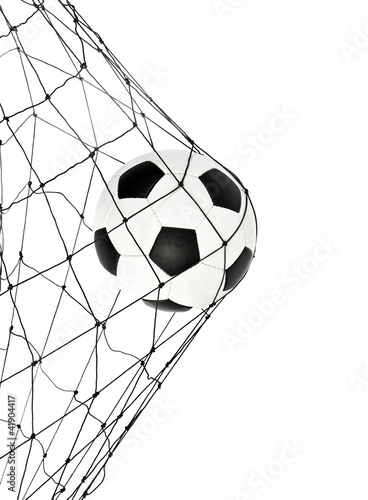This image features a digitally created scene of a soccer ball striking the back of a soccer net. The entire setting is set against a completely white background. The soccer net, appearing off to the left, spans from the upper left-hand corner downward and to the right, with several black lines forming its structure. The net bulges around the center of the image where the black and white soccer ball has presumably just been kicked, capturing the moment of a goal being scored. The ball, which is slightly left of center yet is the focal point, pushes the net outwards. The only other element in the image is a black text watermark that reads "Adobe Stock," located in the bottom left-hand corner. The overall color scheme is strictly black, white, and gray, emphasizing the minimalist yet illustrative nature of this stock photo.